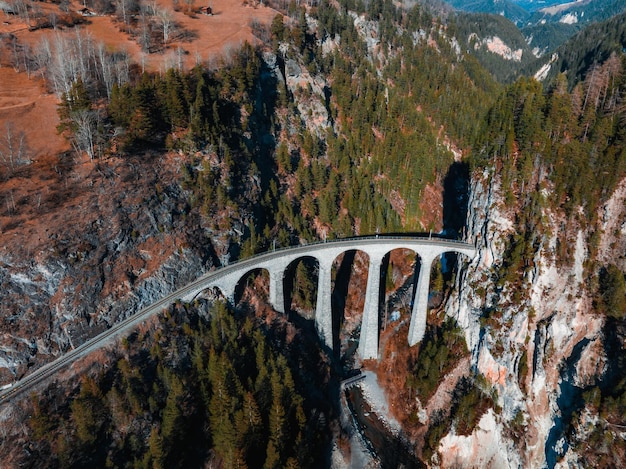This detailed aerial color photograph captures a scenic valley divided by the Landwasser Viaduct Bridge, a towering concrete structure with vertical supports forming elegant arches beneath a gray road. The bridge, which originates from a tunnel carved into the rocky bluff, spans a river dotted with rapids, suggesting a dynamic landscape below. The river valley is flanked by sheer rocky hills on the right, marked by white streaks and crowned with a mix of dead and thriving pine trees, and upward slopes on the left, covered in dark green pine trees and patches of orange clay soil. The sun illuminates the scene, casting reflections on the arches of the bridge, highlighting the realism and depth of the photograph.